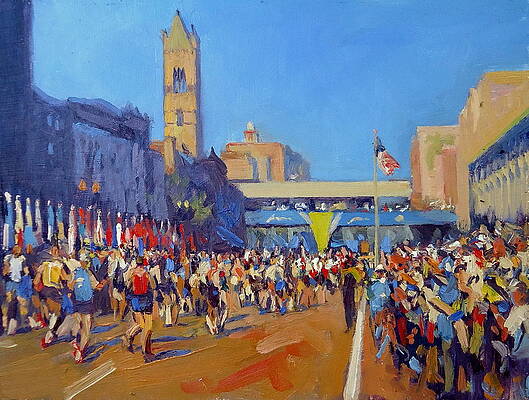This vivid painting captures the energy and vibrancy of a marathon set in an urban environment. The scene is bustling with runners in the forefront, making their way down a brownish-orange, clay-like street towards a distant finish line. This finish line is marked by a blue banner overhead and a vertically descending yellow one. On both the right and left sides of the image, the street is flanked by tall skyscrapers and possibly monumental buildings, suggesting a significant cityscape.

The right side of the painting teems with a lively crowd, cheering the runners on, their enthusiasm almost palpable. Among them, the American flag waves proudly, signifying the national backdrop of the event. This celebratory scene is mirrored on the left side, where more spectators gather, further enhancing the festive atmosphere. Multicolored flags, arranged vertically, lend an international or corporate prestige to the event. A referee stands nearby, ensuring the race is conducted smoothly.

In the middle ground to the left, an old church tower stands prominently behind what appears to be a bridge, indicating the marathon route. The sky above is a clear blue, adding depth and contrast to the bright colors worn by the runners and spectators. Despite a hint of abstraction, the painting's details, from the runners' attire of shorts and T-shirts or tank tops to the diverse crowd, merge into a cohesive and dynamic portrayal of this urban marathon celebration.